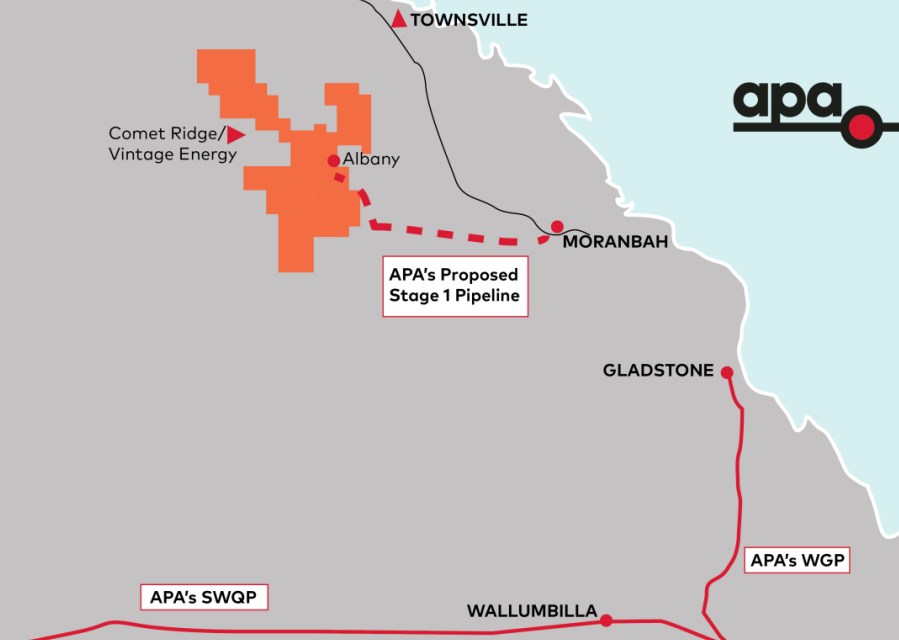This detailed image depicts a meticulously labeled map predominantly shaded in grey, with intricate lines and symbols denoting various key features. At the top right corner, the label "APA" is prominently displayed alongside a distinctive logo comprising a red-filled circle. The map appears to represent an oil pipeline network.

In the center of the image lies a box labeled "APA's Proposed Stage 1 Pipeline," indicating the primary focus of the map. Spreading across the map, a series of interconnected lines paint a picture of this proposed pipeline. A dashed red line traverses from Moranbah to Albany. The map highlights several key locations; notably, it includes labels like Comet Ridge Vintage Energy in an orange-tinted section, further contrasting the generally grey background.

Near the upper right, a red triangle marks the town of Townsville, while further down the coast, Gladstone is clearly annotated with a line proceeding south out of the image, indicating APA's WGP. Another line from Gladstone loops back up to the left, connecting to Wallumbilla and leading to the bottom left corner where APA's SWQP is located. The map is intricately detailed, illustrating a network that connects significant towns and regions, underscoring the reach and complexity of APA's proposed infrastructure.